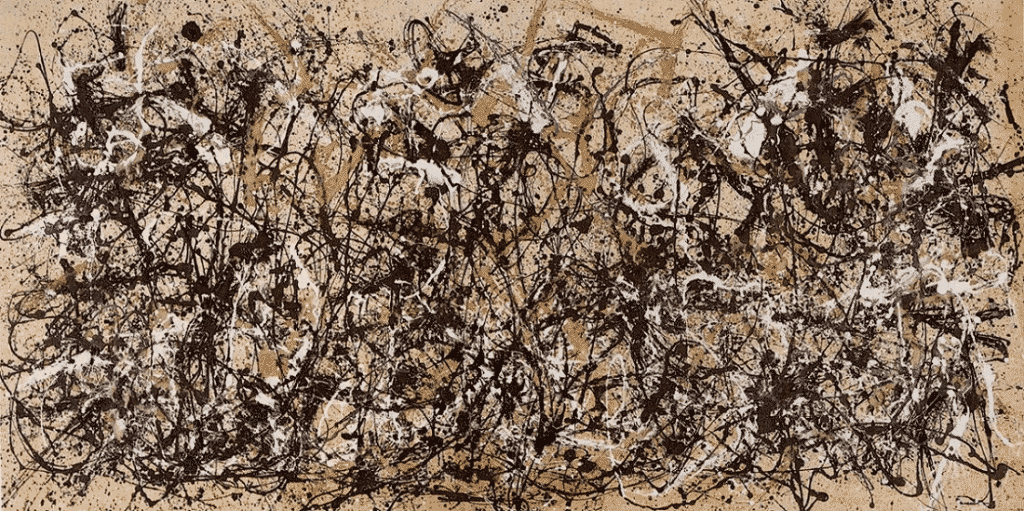This is a rectangular painting with a brownish, cream, or tan background. The painting features an array of colors including tans, browns, blacks, and whites, creating a visually dynamic and modern piece. The background, particularly towards the top and around the edges, is predominantly light brown or beige. The central area is filled with black and white paint splatters, drips, and swishes that give the piece an impressionistic and abstract feel. The paint seems applied in a chaotic manner with no specific pattern or design, resulting in a very messy and busy visual effect. Long, stroked patterns and swirl-like marks are evident throughout, interspersed with occasional straight lines in darker colors. This energetic and staticky arrangement makes the piece feel very modern and might be found on the wall of a contemporary home.